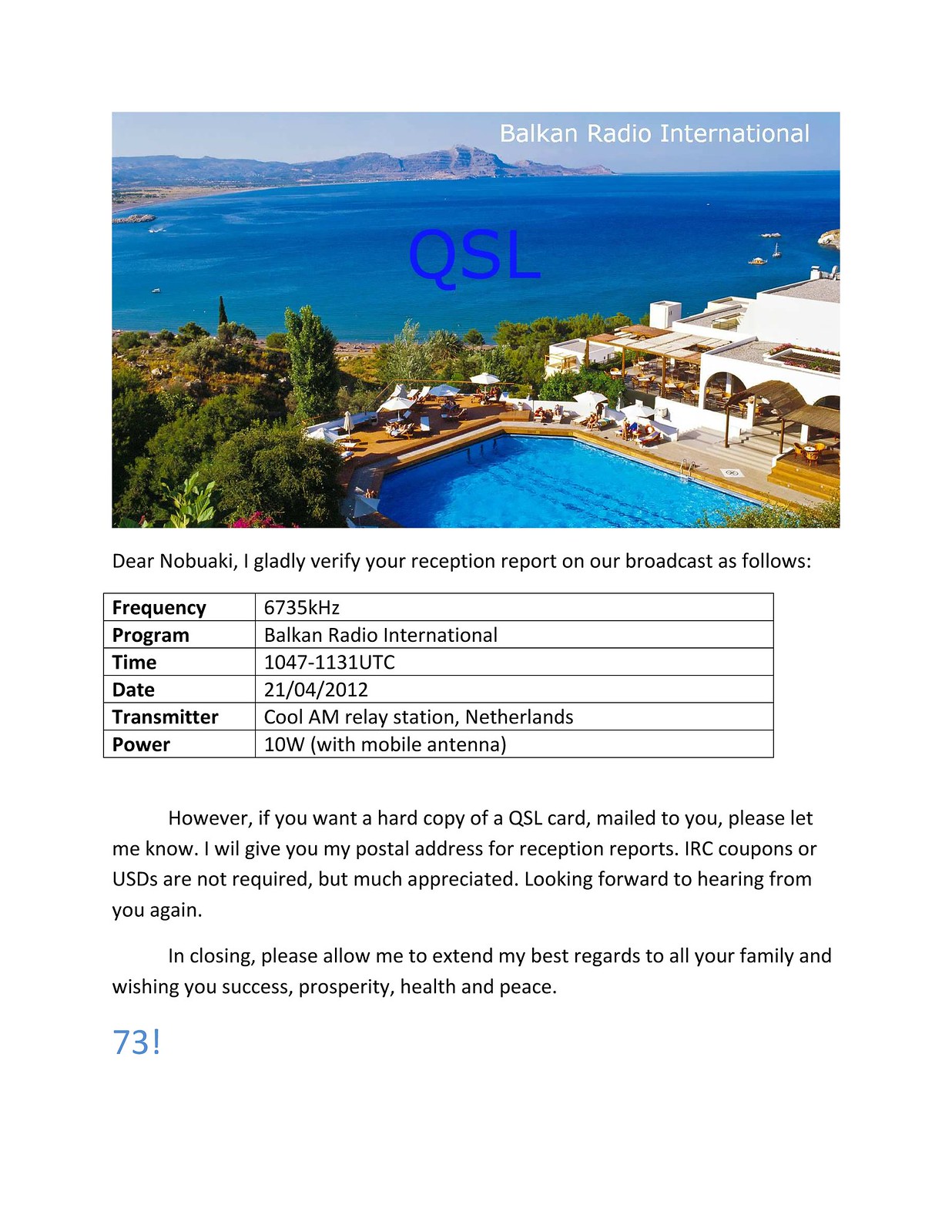The image is a vertically aligned rectangular flyer with a white background. At the top is a larger horizontally aligned color photograph of a scenic resort. The photo showcases a bright blue body of water with mountains in the background and a clear blue sky above. In the foreground, a white resort with a large rectangular swimming pool surrounded by trees, bushes, and white umbrella-shaded tables can be seen. Lounge chairs dot the brown pool deck area. The upper right-hand corner of the photo features the text "Balkan Radio International" in white letters, while the center prominently displays "QSL" in large blue letters.

Below the photograph, the flyer contains black text starting with "Dear Nobuaki, I gladly verify your reception report on our broadcast as follows." This is followed by a two-column, six-row table with bolded headers: Frequency (6735 kHz), Program (Balkan Radio International), Time (1047-1133 UTC), Date (21/04/2012), Transmitter (Kool AM relay station, Netherlands), and Power (10 watt with mobile antenna). 

Further down, the text reads, "However, if you want a hard copy of the QSL card mailed to you, please let me know. I will give you my postal address for reception reports. IRC coupons or USDs are not required but much appreciated. Looking forward to hearing from you again." It concludes with a cordial note, "In closing, please allow me to extend my best regards to all your family, and wishing you success, prosperity, health, and peace." In the lower left-hand corner, stamped in blue, is the number "73!"